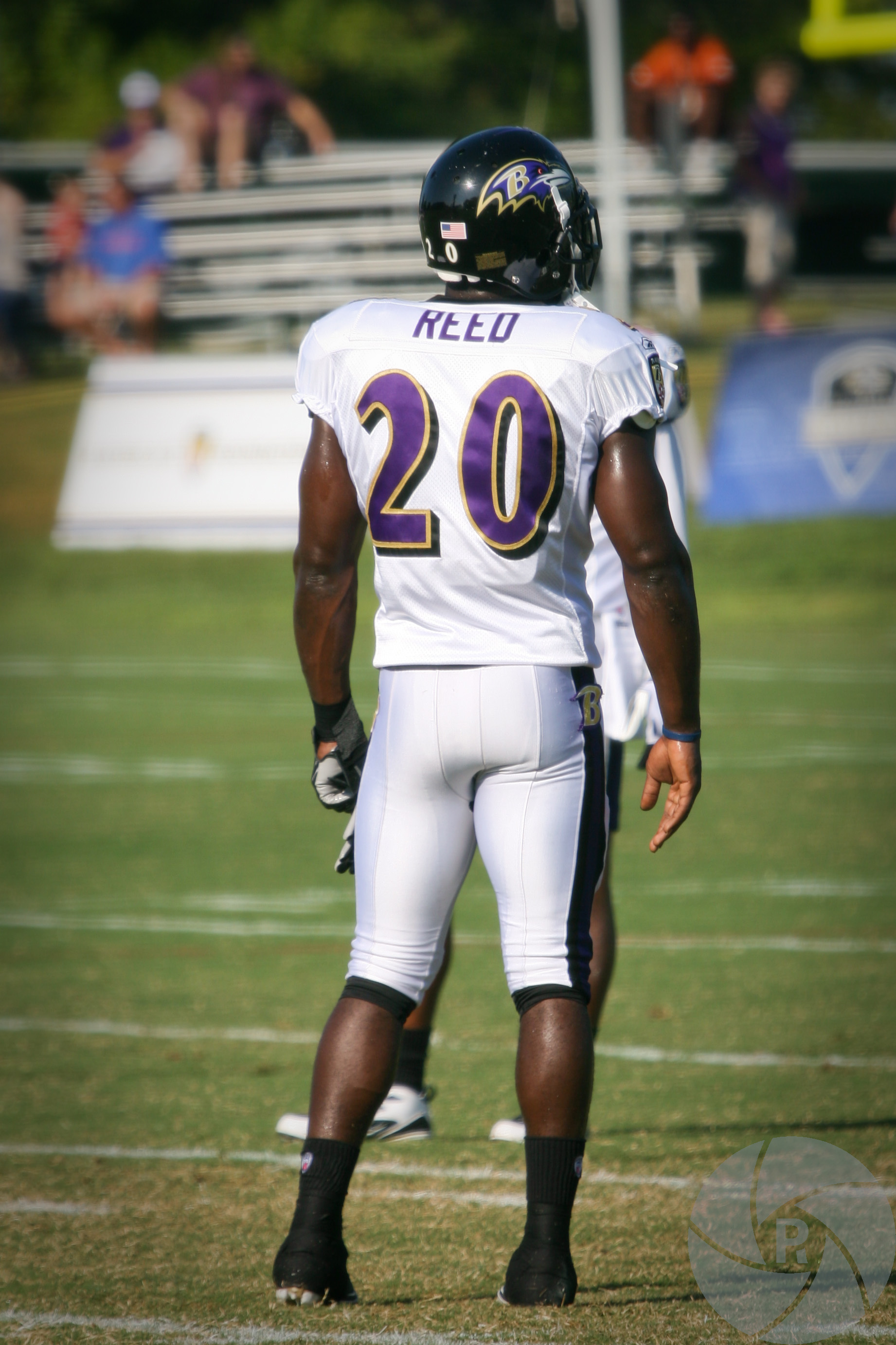The image is a portrait-orientation color photograph capturing the back of a football player standing in the center of a grassy football field during the day. The player, the main subject of the photograph, is wearing a white football jersey with the number 20 on the back, accentuated with a purple color and a yellow drop shadow. The player also wears white pants that are knee-length, featuring black stripes on the sides with a large gold 'B'. Completing his gear, he is clad in black football cleats with white bottoms, black short socks, a dark colored helmet adorned with a graphic of a bird's head and a bold white 'B', and a football armor beneath his jersey. A single glove is on his left hand and he appears slightly sweaty. The football field is marked by short cut grass and multiple white yard lines, with a few dead brown patches scattered throughout. In the background, there are small bleachers with a few blurred spectators—three seated and one standing. Another football player stands mostly obscured by the subject. A semi-transparent, white shutter-like logo with a 'P' is positioned in the bottom right corner of the photograph. The style of the image is photographic representational realism.